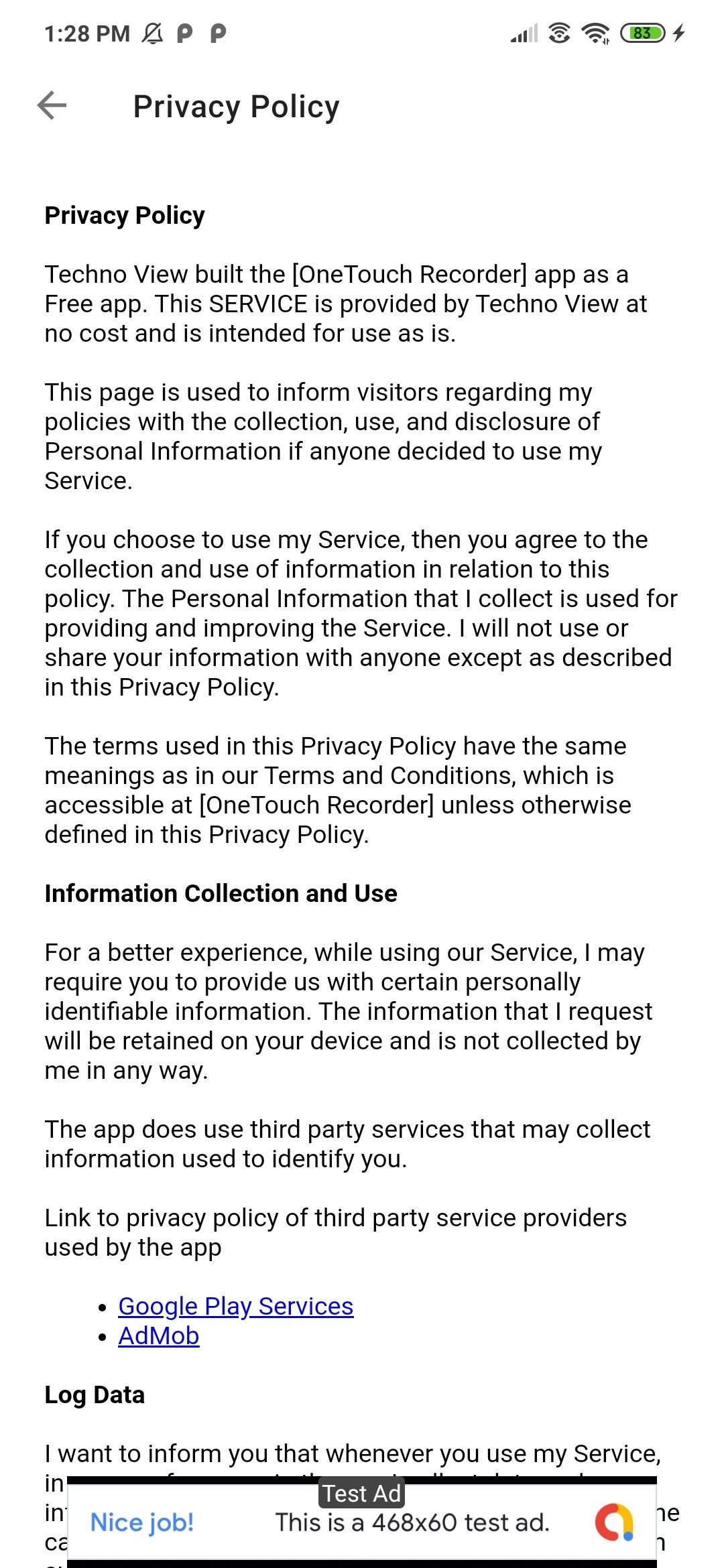This is a cropped screenshot of a mobile phone displaying a privacy policy for an app or game download. At the very top, the screen header reads "Privacy Policy," accompanied by a back arrow on the left side. The main section of the screenshot comprises four paragraphs detailing the privacy policy. Below these paragraphs, a new section titled "Information Collection and Use" is prominently highlighted in bold black font, followed by two paragraphs and a bullet point list that includes hyperlinked terms such as Google Play Services and AdMob.

Further down, the privacy policy continues with another section titled "Log Data," but the content beneath this heading is obstructed by an advertisement. The ad, labeled as a test ad, features the following details: to the left, it displays the message "Nice job," and to the right, it says "This is a 468 by 60 test ad," alongside an icon resembling a rainbow "A".

At the very top of the screenshot, the phone's status bar is visible, showcasing various icons: a lightning bolt indicating charging status, a battery icon, a Wi-Fi icon, and the signal strength icon.